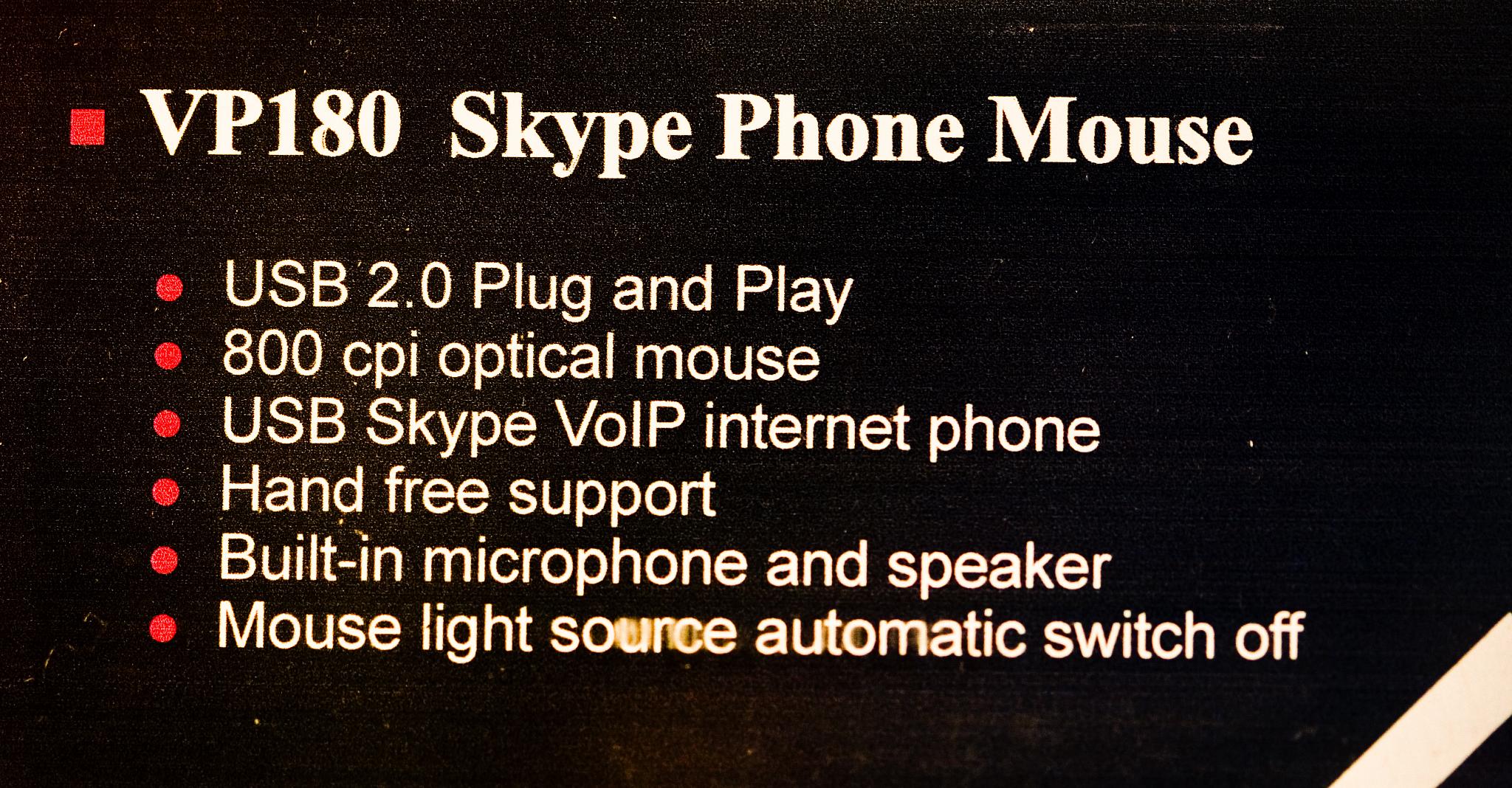This image features a product poster or label, likely part of a presentation or packaging, titled "VP180 Skype Phone Mouse." The design is minimalistic with text organized into bullet points. The main bullet point, denoted by an orange square, prominently displays the product name. Below this, six feature descriptions follow, marked by traditional red circular bullet points. These features include "USB 2.0 plug and play," "800 CPI optical mouse," "USB Skype VoIP internet phone," "hand-free support," "built-in microphone and speaker," and "mouse light source automatic switch off." The text appears slightly aged, with some letters, especially in the last bullet point, showing signs of blurriness. The background is black with white text and might have white specks, resembling dust or scratches on the material.